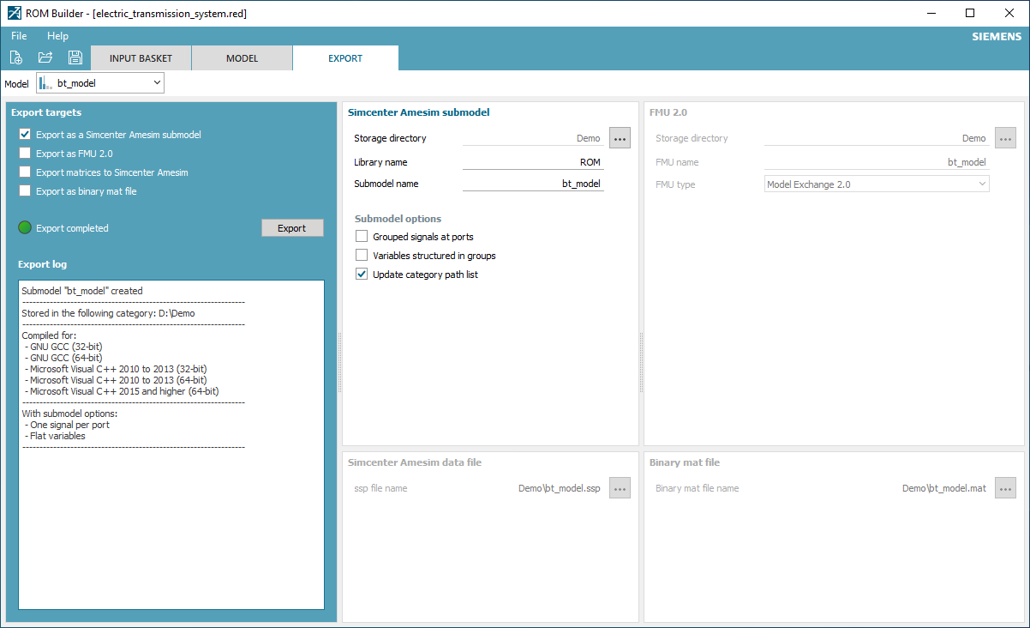This is a detailed screenshot of the ROM Builder application, encapsulated within a Windows window interface. At the very top left corner, the title "ROM Builder" is prominently displayed. Just beneath the title, there is a teal-colored menu bar featuring two options: "File" and "Help". Below this menu, three familiar icons are situated from left to right: a document icon, a folder icon, and a save disk icon.

The interface also comprises four tabs: "Input", "Basket", "Model", and "Export". The "Export" tab is currently selected, highlighted distinctively with white text on a teal background. Directly below this tab, the section header "Model" appears, featuring a dropdown menu labeled "BT_model".

The lower left section of the interface is again in teal, contrasting against a white section to its right. This structured layout ensures easy navigation and user interaction within the application.